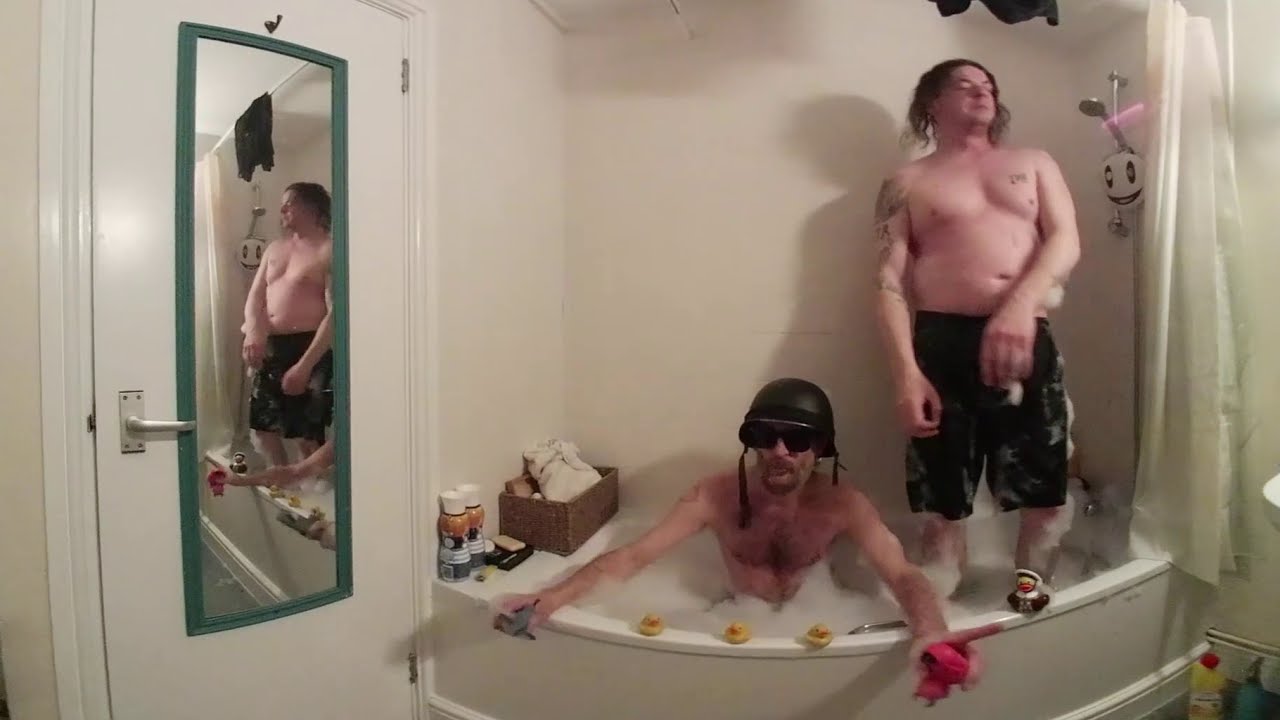This humorous photo captures two Caucasian men, one standing and the other sitting, in a bathtub filled with bubbles, likely having a playful moment. The man on the left is seated in the tub, wearing black goggles, a helmet, and shades. He has dark hair, a mustache with a light stubbly goatee, and is holding a pink toy and a fighter jet toy in his hands. 

On the right, the other man is standing inside the bathtub, wearing black shorts that fall below his knees, displaying tattoos on his arms and chest. His hair is shoulder-length and wavy. He's positioned with one foot in the tub and one foot on the edge, seeming to act as though taking a shower amidst the bubbles.

In front of the bathtub, a line of rubber ducks adds to the playful atmosphere, while on the left side, there are two bottles and a wooden box containing a sack. A door on the left with a green-framed mirror reflects the standing man, showing more of the scene. To the right, a shower curtain, drawn back, exposes the stark white walls of the bathroom and the silver door handle that matches the bathtub's white color.